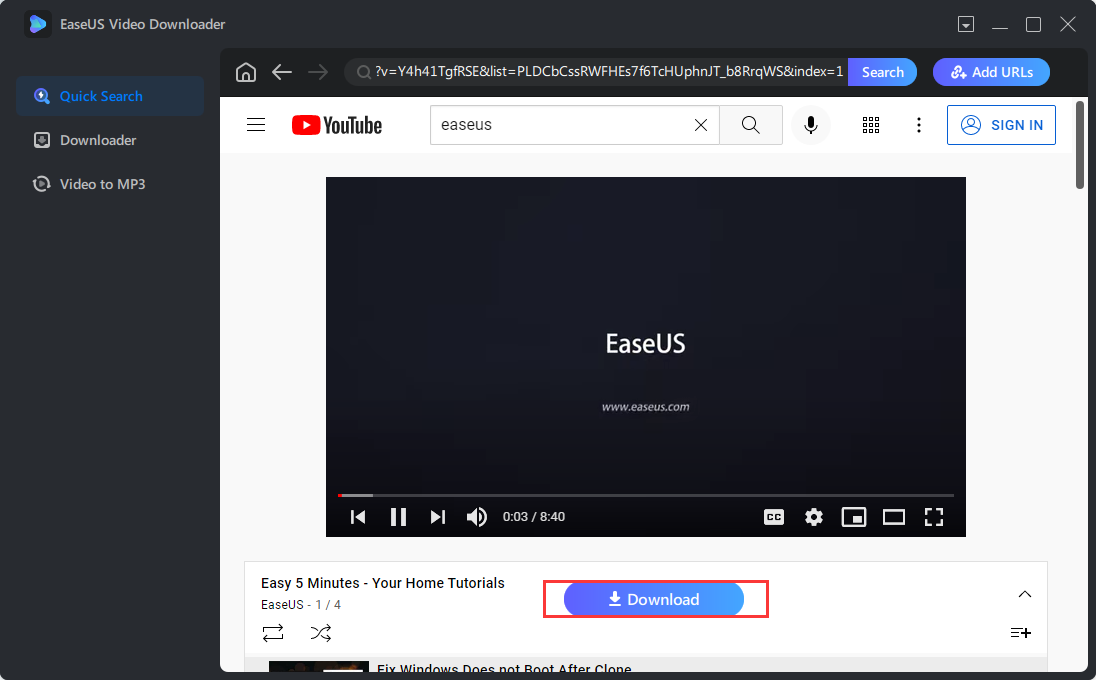The image features a black background with various interface elements displayed prominently. In the upper left-hand corner, there's a small, non-standard shaped square that appears to be a blend of purple and blue tones. Adjacent to this, in white text, it reads "East US Video Downloader."

On the opposite side, there's a white box featuring a downward-pointing white triangle. Below this, a white line leads to an outlined white box containing an "X" symbol. On the left-hand side of the box, the text "Quick Search" is written in blue, followed by "Downloader" in white, and "Video to MP3" also in white.

The center portion of the image holds an open video box. The top section of this video box is black, displaying navigation icons including a white "Home" button, a white left-pointing arrow, a gray right-pointing arrow, and a gray oval containing what seems to be a YouTube link. At the end of this oval, where it transitions into a purplish-blue hue, the word "Search" is written in white.

Below this, there is another purplish-blue oval with "Add URLs" inscribed in white. The remaining section of this box is white, showing three horizontal lines on the left, followed by the YouTube logo inside a red square with a white play button (a triangle).

Further down, there's a white search box labeled "Ease Us" (spelled E-A-S-E-U-S) in blue. Under this section is a black screen displaying the text "Ease Us" in white, along with the URL "www.easeus.com."

The image effectively blends color contrasts and navigational elements typical of a video downloading interface, providing clear indications of functionality and search capabilities.